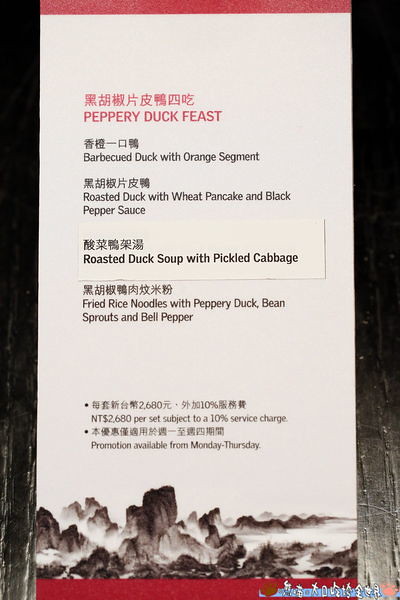The image features a vertically oriented menu flyer with a thin red border at the top and bottom, set against a wooden surface painted black. The paper itself is light gray or white and contains both English and Asian characters (likely Chinese) in various colors.

At the top, within the red border, it says "Peppery Duck Feast" in red, followed by Asian characters in the same color. Below this, in black text, the menu details are listed:

- Barbecued duck with orange segment.
- Roasted duck with wheat pancake and black pepper sauce.
- Roasted duck soup with pickled cabbage (highlighted in a different colored rectangle).
- Fried rice noodles with peppery duck, bean sprouts, and bell peppers.

The lower third of the menu includes pricing details, stating "NT 2,680 per set, subject to a 10% service charge." Below this, it mentions, "Promotion available from Monday to Thursday." Towards the bottom, there's an image of rocks with water crashing against them, bordered by the bottom red line. Something is written in the bottom right-hand corner, though it is not clearly legible. The menu is flanked by visible wood grain on either side, suggesting it rests on a wooden surface.